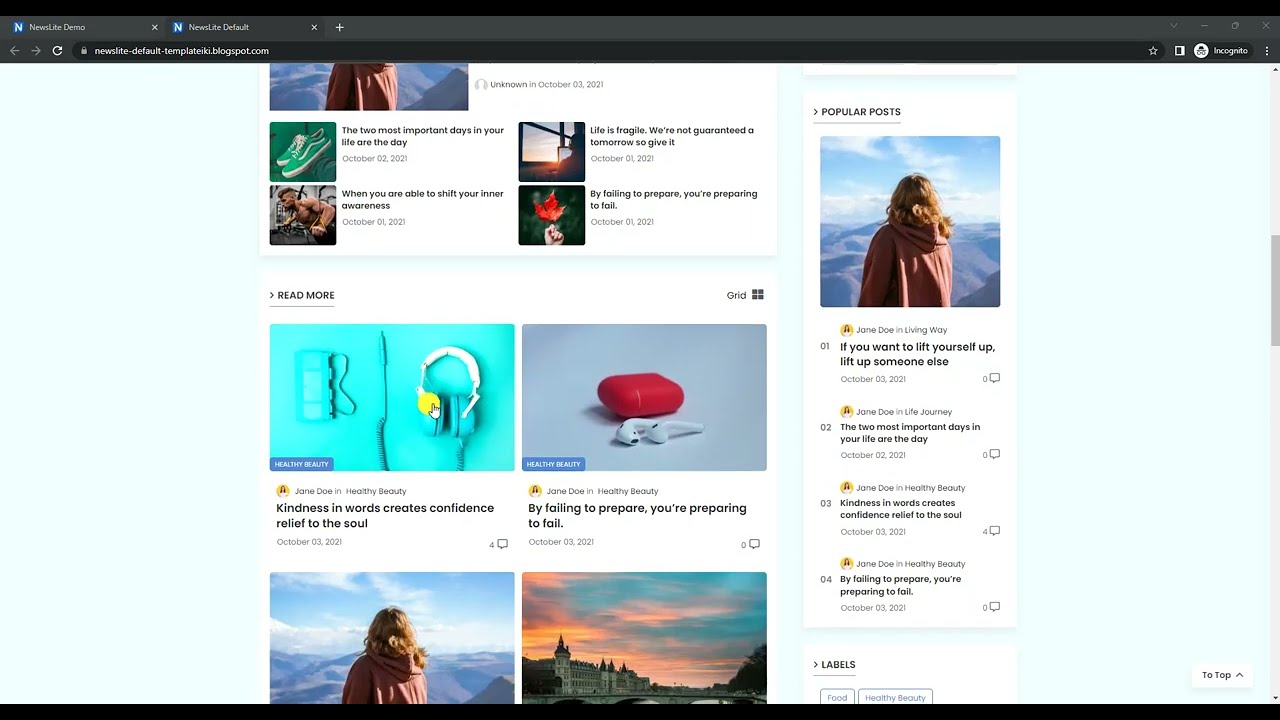The image is of a secondary webpage on a website. At the top, there is a menu bar with folder icons; the left one is labeled "N" accompanied by text, and an adjacent folder also labeled "N" containing some additional details, similar to the previous one. An "X" is located next to both folders. On the right-hand side of this menu bar, there are icons for adding and removing items, a dropdown arrow for the search bar, and a final "X" icon.

Below this menu bar is an address bar equipped with navigation controls, including left and right arrows, a refresh icon, and an address input field flanked by a lengthy search bar. To the right of this search bar are a star icon and an incognito mode indicator.

The main body of the webpage features several media elements, primarily focused on a female figure with her back turned, showcasing her garment. One of the images depicts the sky. There is a section titled "Popular Post" displaying the same woman with her back turned, accompanied by a quote: "If you want to lift yourself up, lift up someone else." Three additional inspirational quotes follow.

In the central area, there are various images, though the person featured in them is partially cut off. A "Read More" link is highlighted, adorned with what seem to be two earbud icons. The woman's image reappears further down, again partially cut off, alongside a reference to a location.